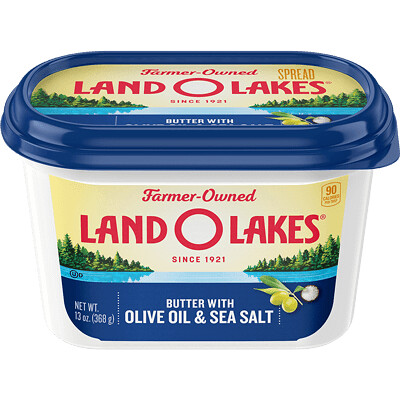This is a professional, close-up photograph of a Land O'Lakes butter tub with olive oil and sea salt. The tub is rectangular, plastic, and white, viewed straight on. The lid has a blue edge with the text "Farmer-Owned Land O'Lakes Spreads since 1921" in red. The image on both the lid and the front label features a picturesque outdoor scene: a clear blue lake surrounded by pine trees, and a yellow sky in the background. The label includes multiple details: "Butter With Olive Oil and Sea Salt" written in white text on a blue background, a drawing of two olives on a branch, and a pile of salt. Additionally, the label indicates a net weight of 13 ounces (368 grams) and mentions "90 calories per serving" in the upper right corner. The consistent design elements on the lid and label provide a uniform and appealing presentation.